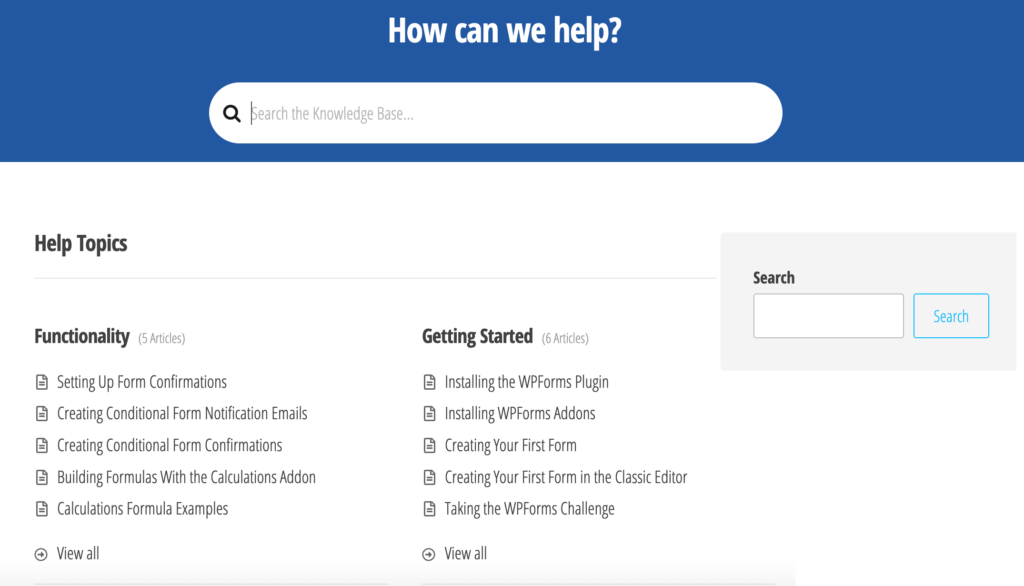The image features a support page layout with a predominantly white background and a blue header. At the top of the image, centered within the blue header, white text reads "How can we help?" Directly below is a gray search bar containing the placeholder text "Search the knowledge base..." 

On the left-hand side, there's a section titled "Help Topics" in black text. Beneath this heading, a series of help topics are listed in gray text, including:
- Setting Up Form Confirmations
- Creating Confidential Form Notification Emails
- Creating Confidential Form Confirmations
- Building Formulas with Calculations Add-On
- Calculations Formula Examples

The list ends with a "View All" option in gray text.

On the right-hand side, another section entitled "Getting Started" in black text is presented. Underneath this heading, in gray text, there are additional help topics:
- Installing WPForms Plugin
- Installing WPForms Add-Ons
- Creating Your First Form
- Creating Your First Form in the Classic Editor
- Taking the WPForms Challenge

This list also concludes with a "View All" option in gray text.

Towards the bottom right of the image, there is a small blue box with the word "Search" in black text. Directly below this box is a white input field where users can type search queries. Further right is a blue button with blue text that also reads "Search". The page has been described in detail, covering all the elements that are present.